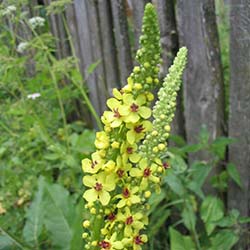This image captures a picturesque outdoor scene in a garden. At the very forefront, two tall green stems, reminiscent of corn stalks, stand prominently. These stems are adorned with several small yellow flowers, each boasting a vivid orange-red center. The flowers cluster densely along the stalks, with one stalk having six flowers and the other six, making a total of twelve. The image's main focus is on these flowering stalks, which appear to rise nearly to the top border of the picture. In the background, an old, weathered wooden fence with brown, vertically arranged slats provides a rustic backdrop, indicating that it has been standing there for quite some time. The fence slats do not touch, leaving small gaps between them. To the left of the flowering stalks, diverse foliage and wildflowers, including white blossoms, contribute to the lush greenery. The mixed variety of leaves and plants complements the garden's natural and slightly untamed appearance. The scene exudes a serene, slightly whimsical charm, accentuated by the simple yet vibrant details of the flora.